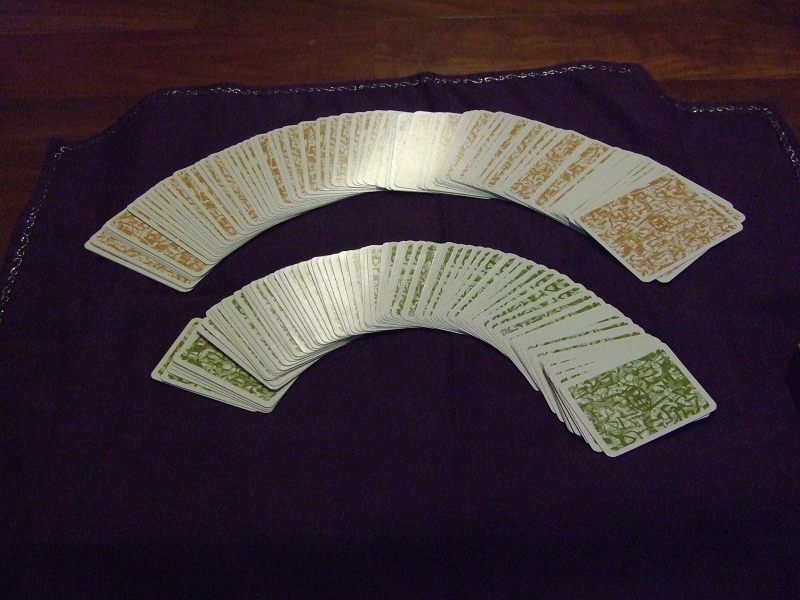The rectangular photograph showcases a visually captivating arrangement featuring two decks of playing cards fanned out against a rich backdrop. In the center of the image, both decks are meticulously fanned with the curved sections gracefully pointing upwards. The deck at the bottom displays an intricate green line design, framed by a clean white border. In contrast, the deck above it boasts an identical line pattern but in a vibrant orange hue, also bordered in white.

These decks are elegantly positioned on a square piece of purple cloth, decorated with a subtle silver border. The fabric is notably wrinkled and folded, with prominent fold lines visibly running from the top center to the bottom. The layout of the cloth appears casual and natural, with its edges noticeably out of frame at the bottom right, bottom left, and bottom sections of the image.

Surrounding this central display, the cloth rests on a dark brown wooden surface composed of distinct wood planks, adding a rustic texture to the composition. The interplay of the colorful cards, purple cloth, and wooden background creates a rich and detailed visual narrative.